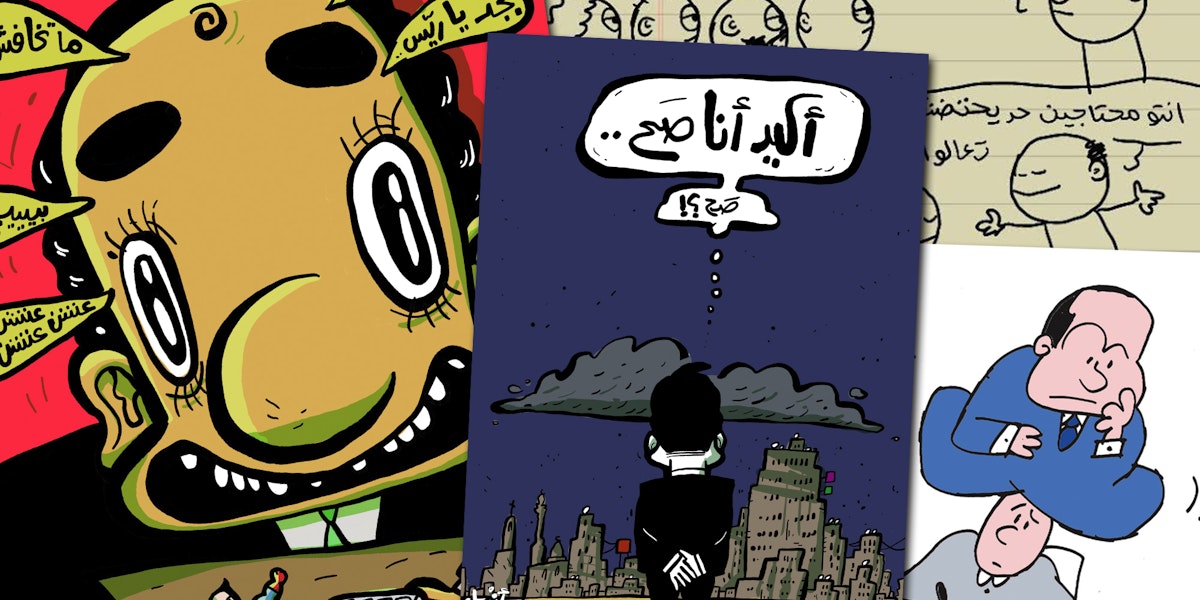The image is a small horizontal collage of stylized cartoon illustrations of people, presented side by side. The left part of the collage features a large, close-up pop art depiction of a man's head with exaggerated, beady vertical eyes and a wide-open black mouth, revealing white teeth. The man has a weird facial expression that is very cartoonish and over-the-top, with Arabic or Middle Eastern script written on the image. In the background, there's a cityscape under a cloudy sky. This section also includes a simple sketch of a redheaded man wearing a gray shirt.

The central part of the collage shows a man against a dark blue backdrop, with his hands clasped behind his back. He appears to be looking over a city, suggesting a contemplative mood. This figure is depicted from behind within a purple square.

The right section of the collage features a unique and surreal composition—one man in a blue suit jacket with cufflinks, sitting in a meditative pose on top of another man's head. The man with the cufflinks seems to be in deep thought. Additionally, the top right corner of this section includes simple pin drawings on what appears to be a yellow steno pad, showing round heads with varied facial expressions. Thought bubbles with indistinct text and squiggles emerge from the characters' heads, adding to the whimsical and illustrative nature of the artwork.